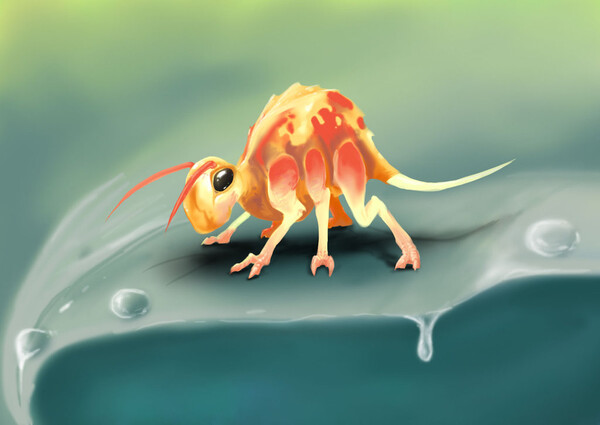The image is a computer-animated digital artwork, styled to resemble watercolor animation, adorned with smooth and vivid details. Set against a fuzzy green background that evokes a forest or woodland scene, it features a single leaf in the foreground, glistening with dewdrops and moisture dripping off its edge. Resting on this dewy leaf is an intricate, cartoonish insect. The creature, poised as if about to jump, has a blend of bright hues: its arched back is adorned in shades of orange, yellow, red, and light brown, seamlessly graduating into its six legs that transition from red to yellow and white. The insect’s long yellow tail, reminiscent of a rat’s, points to the right, while its red antlers or antennae extend forward. It possesses large, expressive black eyes that appear to stare directly at the observer, imparting a sense of curiosity and animation. The detailed rendering of the insect and its poised stance creates a dynamic and engaging scene, capturing a moment of stillness and imminent motion.